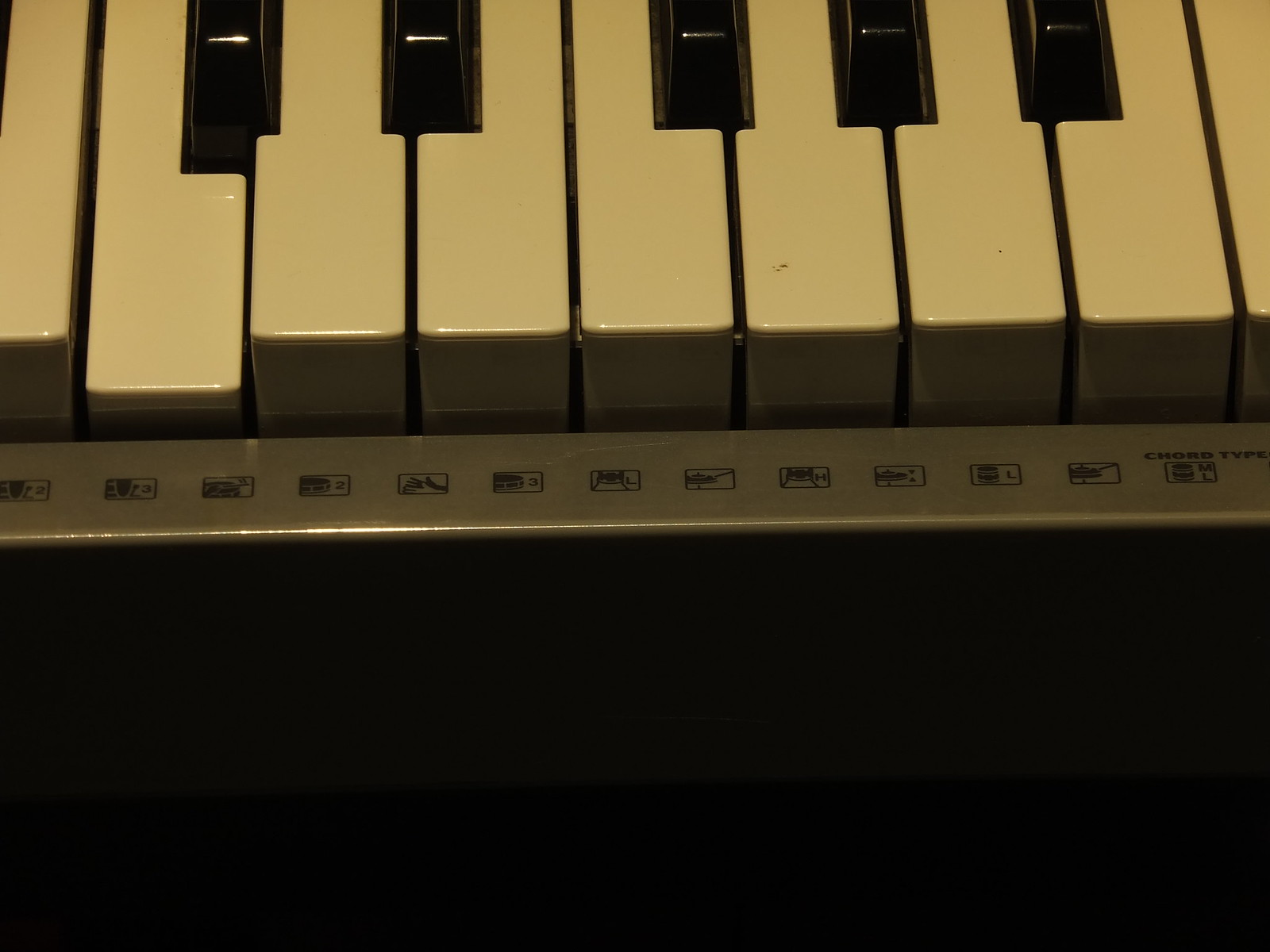This image is an up-close, detailed view of a keyboard, likely an electronic one due to the metallic or plastic-looking gray frame. The photograph captures nine white keys, with seven full keys and one partial key on each end, along with five black keys in the background. The second white key from the left is slightly depressed, indicating a note being played. Below the white keys, there is a strip with small squares containing unreadable symbols, potentially note names or chord types, with the words "Chord Type" clearly visible in the top right of this strip. The lighting in the image seems dim, casting a yellowish hue over the normally white keys. The bottom of the image fades into pure black, giving no further context about the surrounding environment.